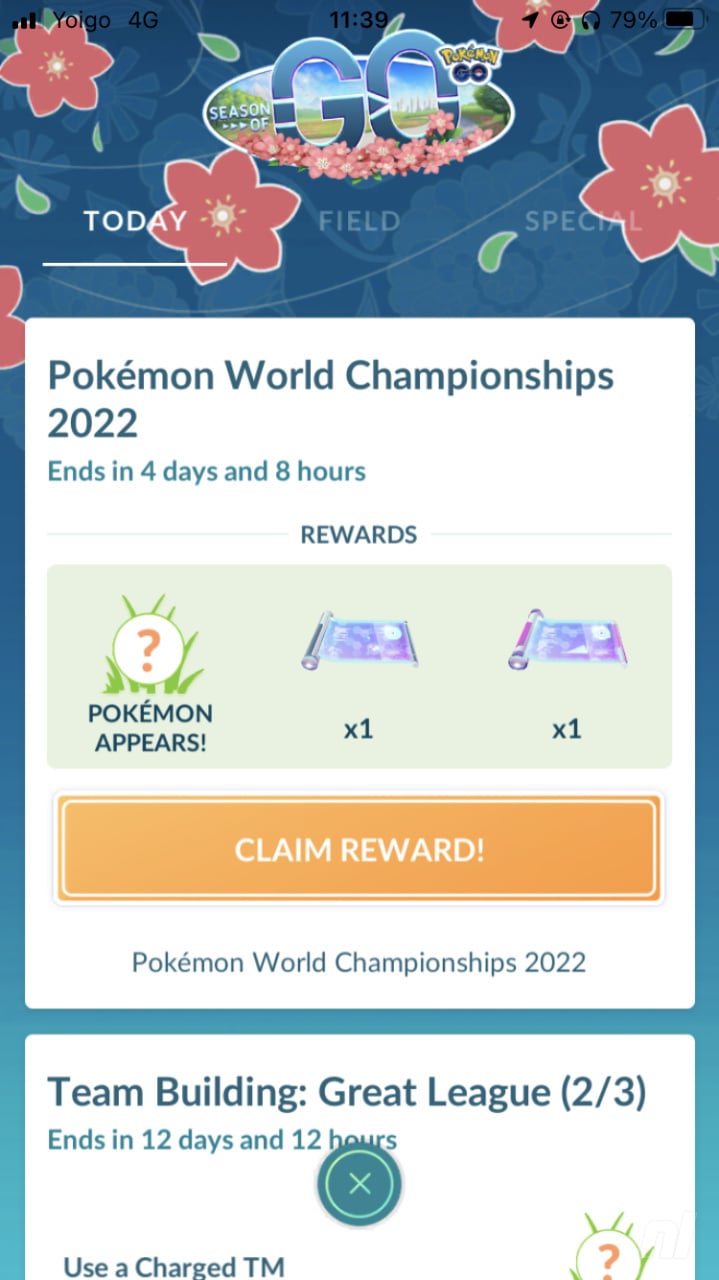The image showcases a smartphone screen displaying the Pokémon Go app. Prominently featured is a notification flyer announcing an in-game event. At the top of the screen, the word "Go" is visible along with the phrase "Season of Something." There are three navigational tabs labeled "Today," "Field," and "Special." The device's status bar indicates it is 11:39, connected to the Yolgo 4G network, and has a battery level of 79%.

Below the event header, the flyer promotes the Pokémon World Championships 2022, noting that the event ends in four days and eight hours. The rewards for participating include a Pokémon encounter and several other undisclosed items. A "Claim Rewards" button is also present, along with a mention of "Team Building: Great."